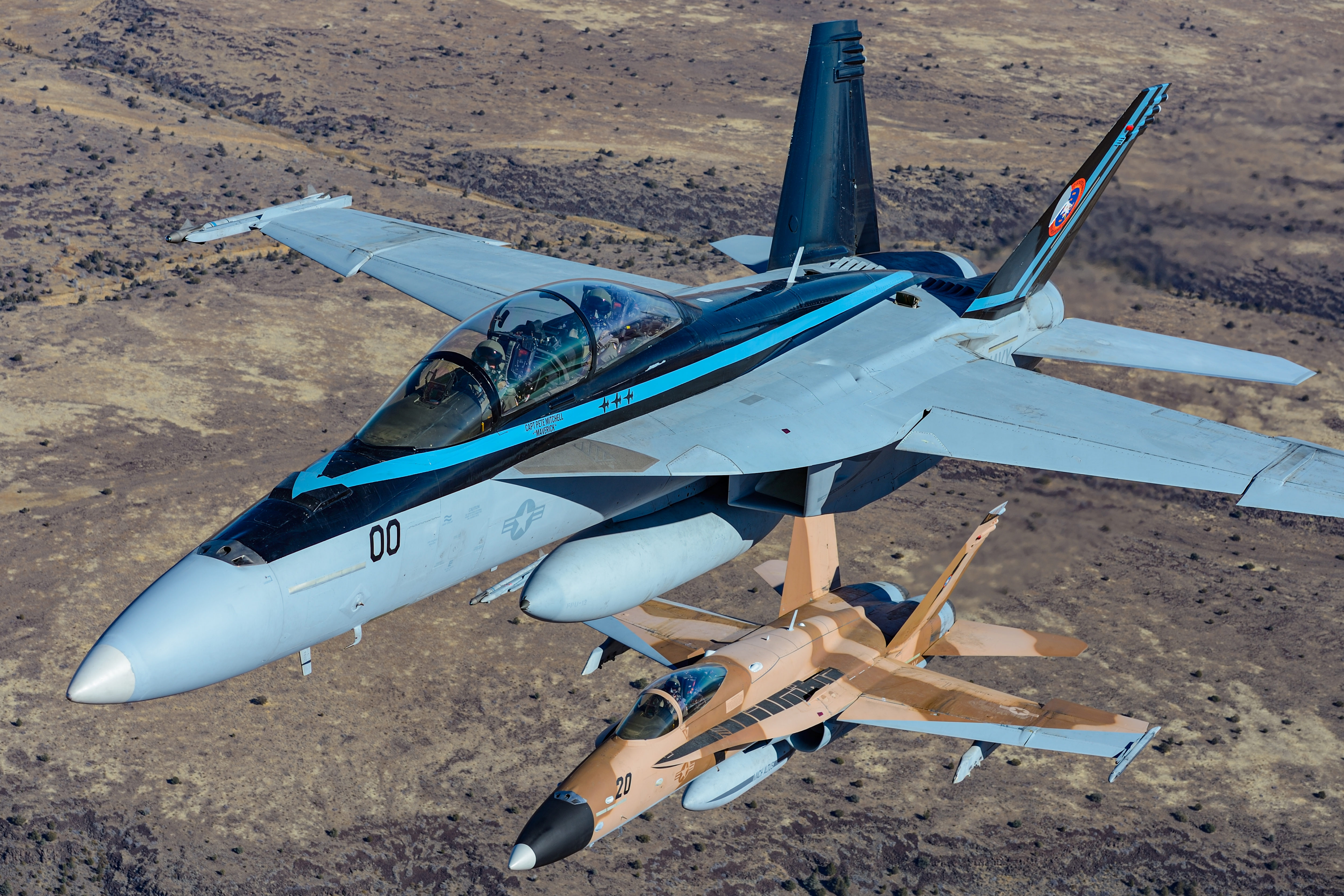This aerial photograph captures two fighter jets flying over a barren, desert landscape. The jet in the foreground is painted a striking blue-gray and features a glass-enclosed cockpit housing two pilots—one wearing dark goggles and another seated behind. This aircraft also bears the number "00" and has a light blue stripe running beneath the cockpit along with dark blue stars. Under its wings, you can see missile or fuel tank-like attachments, and a distinguishable intake scoop below. Additionally, there is a large missile carried underneath. Below the prominent jet, a second, similar jet is visible, painted in desert camouflage shades of brown and gray. This camouflaged jet, which carries just one pilot and bears the number "20," also has a missile attached underneath. The stark contrast between the sleek blue-gray jet and the rugged desert camouflage plane against the arid backdrop makes for a compelling military scene. The photograph seems taken from another aircraft or drone, capturing the high-altitude operation in a remote, desolate area likely resembling the Middle East or the Arizona desert.